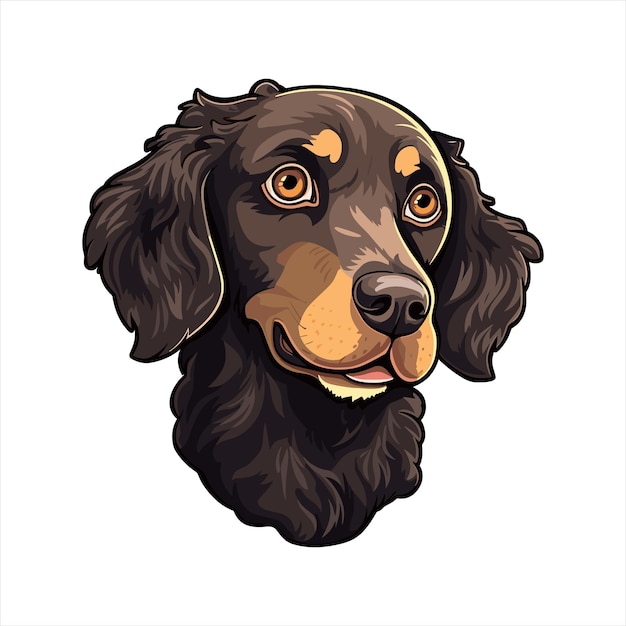This digital sketch depicts a young spaniel-like dog, head viewed from the neck up on a white background. The dog has medium-length, predominantly dark brown fur with subtle variations in hue. The fur is notably fluffy and curled on the ears and neck, whereas it is shorter and smoother on the head and muzzle. The dog's eyes, a striking golden amber with dark pupils, are accented by two tan splotches above them, resembling eyebrows. The muzzle exhibits a tan coloration that contrasts with the darker brown fur around its face, transitioning into a light brown hue towards the snout. The nose is a soft brown, and a few short whiskers are visible on the muzzle. The dog's mouth is slightly open, revealing a glimpse of its pink-red tongue. The dog gazes to the left side of the image, offering a profile that captures its gentle and youthful demeanor. Overall, the image is a colored drawing rich in detail, giving life-like texture and depth to each element of the dog's appearance.